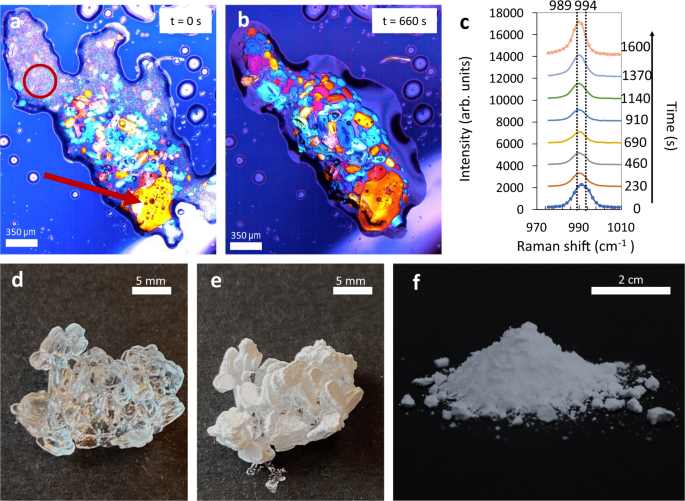This image presents a detailed scientific study of crystallization over time and its effects on surrounding materials, shown in six labeled panels (A-F).

- **Panel A:** Displays a microscopic, blue-tinted image of an amorphous, liquid-like cell with multicolored elements (light blue, yellow, red, etc.). The panel is titled "T = 0s" indicating the initial observation time. A 350-micron scale bar is included for reference.
- **Panel B:** Shows a subsequent microscopic view at "T = 660s," where the cell has darkened and the internal colors have intensified (e.g., yellow regions turning bright orange, pale blues turning deep blue). This also includes a 350-micron scale bar.
- **Panel C:** Features a graph titled with "Raman Shift" (970-1010 cm⁻¹) on the x-axis and "Intensity (ARB Units)" on the left y-axis, with "Time (s)" scaling from 0 to 1600 on the right y-axis. The graph contains eight multi-colored lines, illustrating intensity changes over time peaking in the middle.
- **Panel D:** Shows a crystal structure, appearing translucent and bubble-like, with a 5-millimeter scale bar against a dark gray background.
- **Panel E:** Depicts another crystal, less transparent and appearing more solid and chalky, similarly labeled with a 5-millimeter scale bar and presented on a dark gray background.
- **Panel F:** Illustrates a pile of white powder on a black background, marked with a 2-centimeter scale bar.

Each panel provides a snapshot of the material at different stages or magnifications, combining microscopy, time-lapse imaging, and spectroscopy to offer a comprehensive overview of the process.